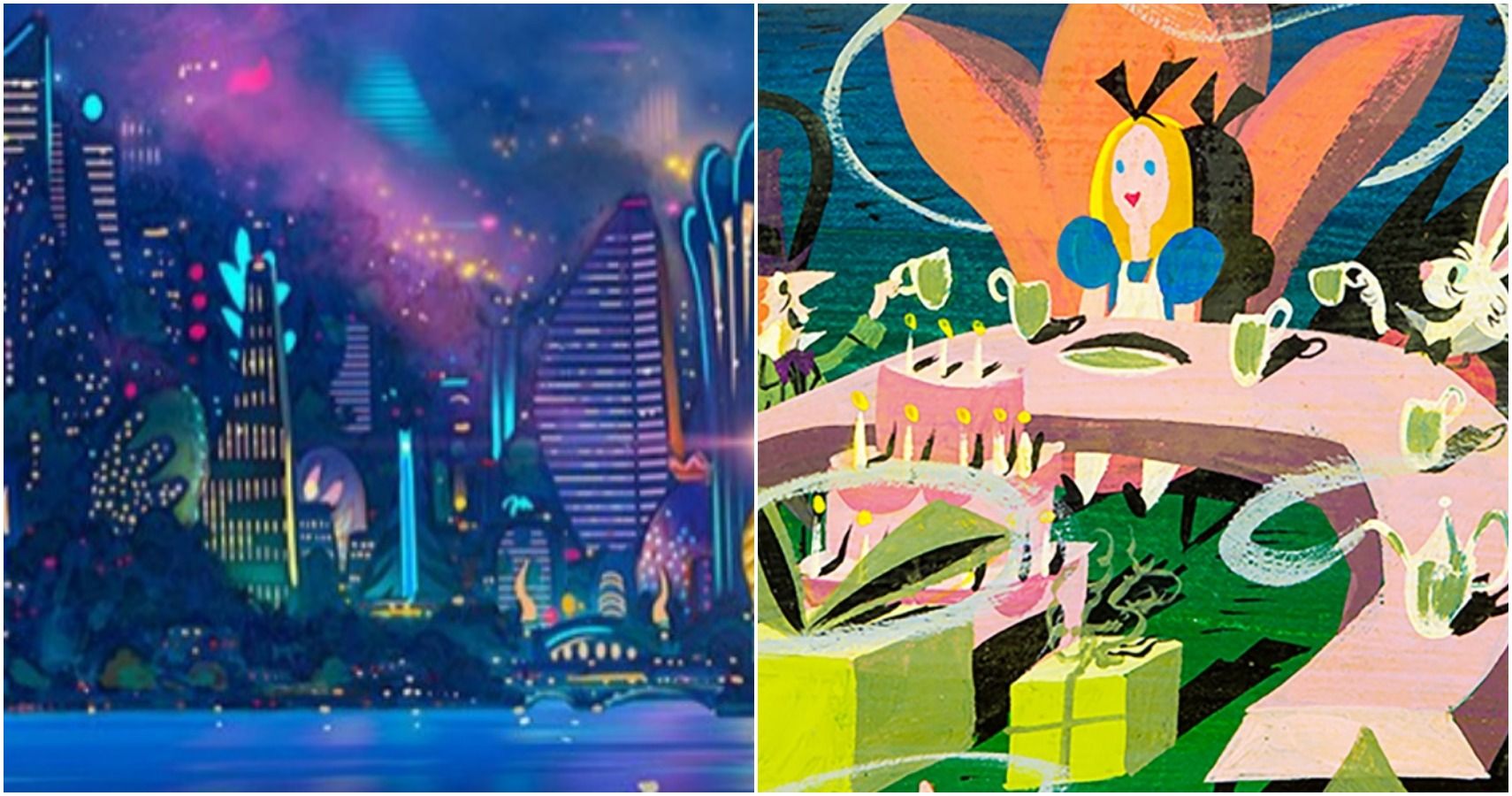This vibrant, stylized image is divided into two distinct sections by a thin vertical white line. The left side presents an abstract cityscape bathed in nocturnal hues of blue, purple, and green, accented by splashes of yellow light. Tall, varied skyscrapers elegantly descend in height diagonally from left to right, transitioning down to smaller central buildings. A prominent, uniquely leaf-shaped purple skyscraper stands out, with its rounded base and pointed top, flanked by green bushes and a small blue bridge. At the bottom, the water body—reflecting the city lights—creates a dynamic interplay of blue and purple tones, adding to the scene's surreal ambiance. The sky above exhibits a mesmerizing cosmic aurora borealis effect with streaks of purple.

The right side brings to life a whimsical tea party from Alice in Wonderland, rendered in a playful, minimalist cartoon style. Central to this scene is Alice, characterized by her iconic yellow hair, large black bow, and wide blue dress, seated on a grand green throne-like chair. She faces forward, surrounded by an intimate gathering. The Mad Hatter, adorned in a purple hat and green suit, sits to her right, offering a cup of tea, while the White Rabbit, in a red suit with a bow tie, mirrors the gesture on her left. A pink boomerang-shaped table stretches across the foreground, laden with tea party staples, including green teacups, a tiered pink cake with candles, and two large green-wrapped presents. The entire scene bursts with vivid greens, pinks, and yellows, encapsulating the fantastical essence of the Wonderland narrative.